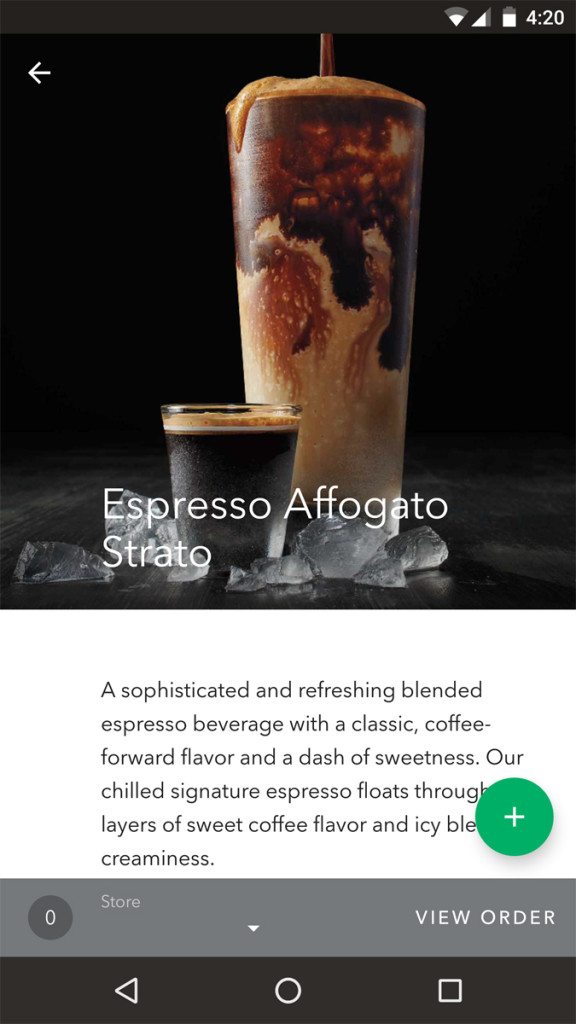The image, likely taken on a smartphone, showcases a sophisticated coffee beverage at precisely 4:20 PM, as indicated by the device's clock. At the center of the image is a sleek black box containing a large clear glass filled with an Espresso Affogato Strato. The beautifully blended coffee in the glass has a syrup layer on top that gracefully drips down, creating intricate patterns of darker and lighter shades. A clear straw emerges from the frothy concoction, which overflows slightly, adding to the drink's allure.

Next to the main drink, there's a small, clear glass of concentrated espresso. Below the glasses is a descriptive text that reads: "A sophisticated and refreshing blended Espresso beverage with a classic coffee-forward flavor and a dash of sweetness. Our chilled signature Espresso floats through the layers of sweet coffee flavor and icy blend creaminess." 

In the background is a gray-toned image with a gradient from dark gray at the top to black at the bottom. The word "Store" is prominently displayed, accompanied by drop-down options to view orders. The current order count is zero.